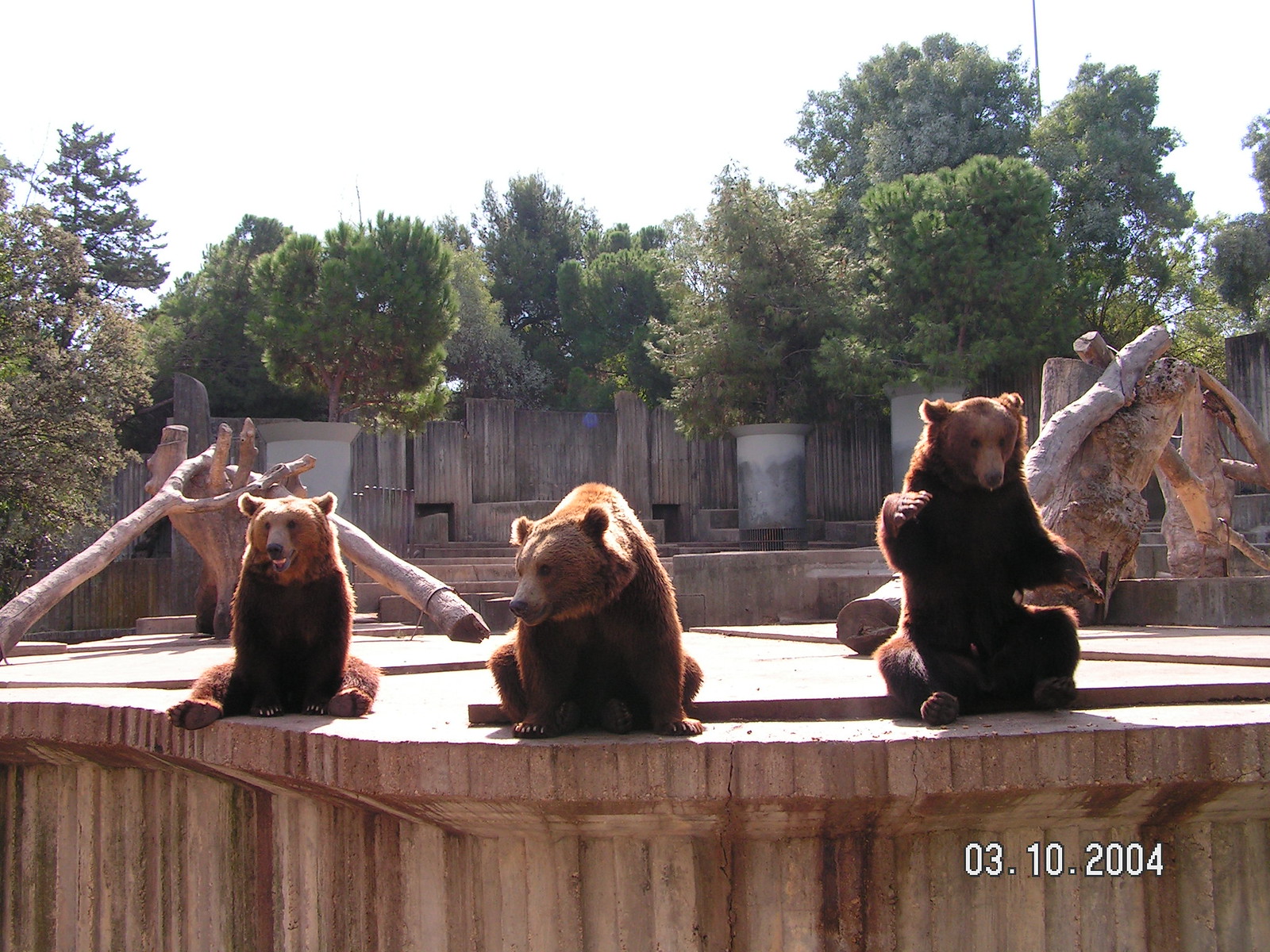The image, taken on March 10, 2004, captures a bright, sunny day at a zoo. It features three brown bears sitting on a stone and cement platform within their enclosure. The enclosure itself is surrounded by a wooden and cement barrier, with trees and logs designed for the bears' exercise in the background. The three bears appear to be a family, with two larger bears potentially the parents and a smaller cub. 

The bear on the left is sitting on its hind legs, with its front feet forward and its arms raised slightly in what appears to be a playful manner. The middle bear, also sitting but positioned more forward on all fours, looks slightly to the left. The bear on the right sits upright on its haunches with its arms spread wide. All three bears' coats gleam brightly under the sunlight, suggesting a clear, bright day despite the cloudy sky. The scene gives an overall impression of a peaceful moment, with the bears seemingly relaxed and content in their environment.